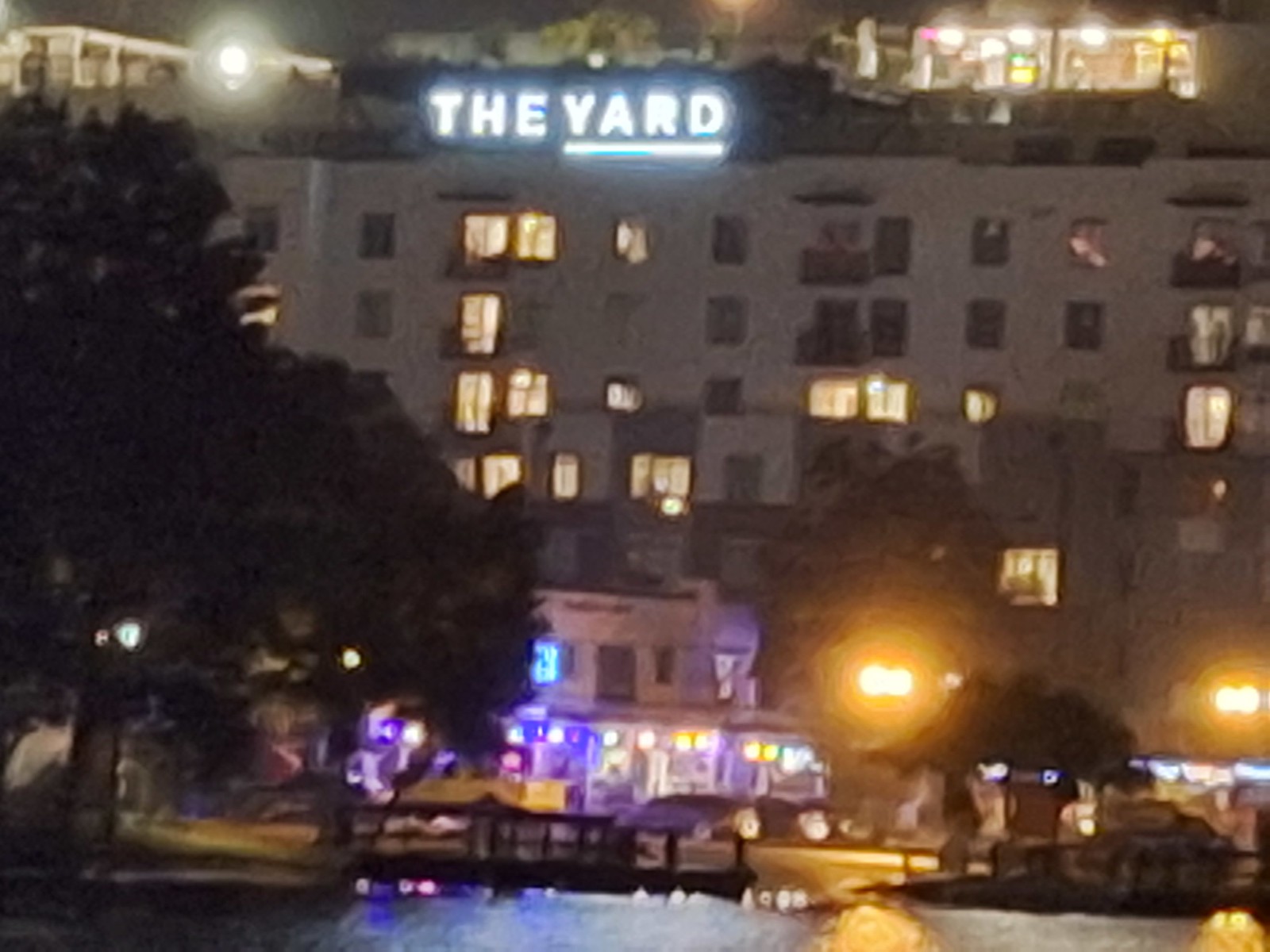In this outdoor photograph, we are introduced to a prominent large structure that dominates the frame. Despite the blurriness, the building appears to be a light-colored establishment, potentially a hotel, as indicated by a neon sign atop it that reads "The Yard." At street level, illuminated shopfronts are discernible, adding to the bustling ambiance of the scene. The presence of parked cars along the street suggests an active urban setting. Trees are visible towards the base of the image, which, alongside hints of a small water body—either a stream or a canal—enhances the locale's natural charm. The overall composition hints at a lively yet serene environment, marrying architectural grandeur with urban vitality and natural beauty.